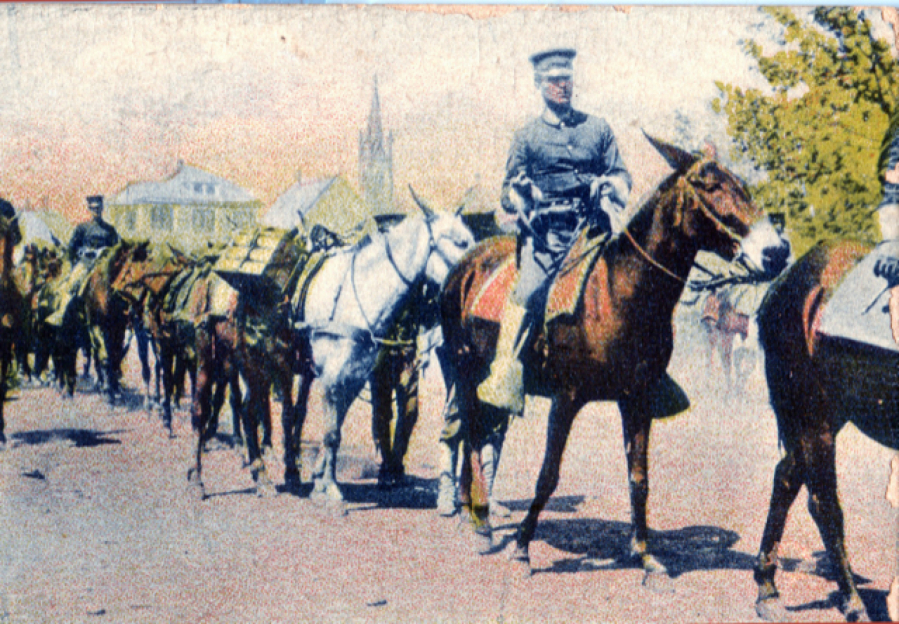This image appears to be an old, damaged photograph or possibly a painting, taken during the daytime in a small village. The scene features a prominent, tall tower towards the middle left-hand side and a modest, two-story house further left. The background includes buildings with a muted peach and yellow hue topped with white roofs. Notably, there's also a church steeple visible.

In the foreground, a line of horses stretches across, some bearing soldiers in gray hats and buttoned-up shirts. One conspicuous soldier rides a brown horse with a white muzzle. Following behind are several pack mules carrying yellow boxes, indicative of supplies. The horses and mules move in a procession led by soldiers, suggesting they might be headed to or returning from a military expedition. To the right background, lush green trees add to the pastoral yet historical ambiance of the scene.